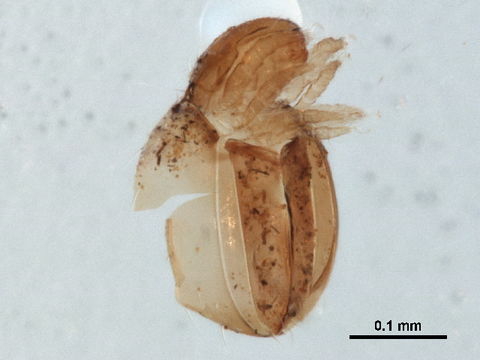This image, set against a white background, features a highly magnified, light to brownish-tan translucent object that measures merely 0.1 millimeter, as indicated by the black, underlined writing in the bottom right-hand corner. The image suggests intricate details reminiscent of either biological or textured material. The object has the appearance of a tied ribbon or a small insect, such as a flea or tick, due to its segmented, possibly leg-like structures and an identifiable head and abdomen. The texture bears semblance to a banana peel or potato skin, hinting at a possibly organic origin. Given the microscopic scale, we observe details that depict a significant degree of magnification, revealing aspects not discernible with the naked eye.